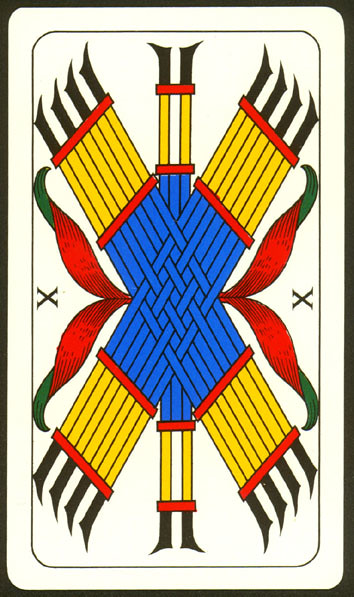This image showcases the back of a playing card featuring an intricate and vivid design. The card is bordered by a black rectangle, with a white rectangle inside of it that has rounded corners. The central graphic consists of a prominent cross-shaped design, formed by two wide crosses interweaving with each other. This arrangement is set against a vertical strip that runs up and down the card.

The interwoven crosses have a detailed color scheme: the central parts of the crosses display a striking blue, surrounded by a red border, followed by a yellow section, and finishing with another red border. Extending outward from each arm of the cross are black blade-like elements, with a similar but narrower shape positioned in the middle.

The card's edges are adorned with floral motifs, resembling red flower petals or leaves with one side painted red and the other green. Positioned between these floral elements on each side of the card are small 'X' shapes, adding to the overall ornate and symmetrical design.